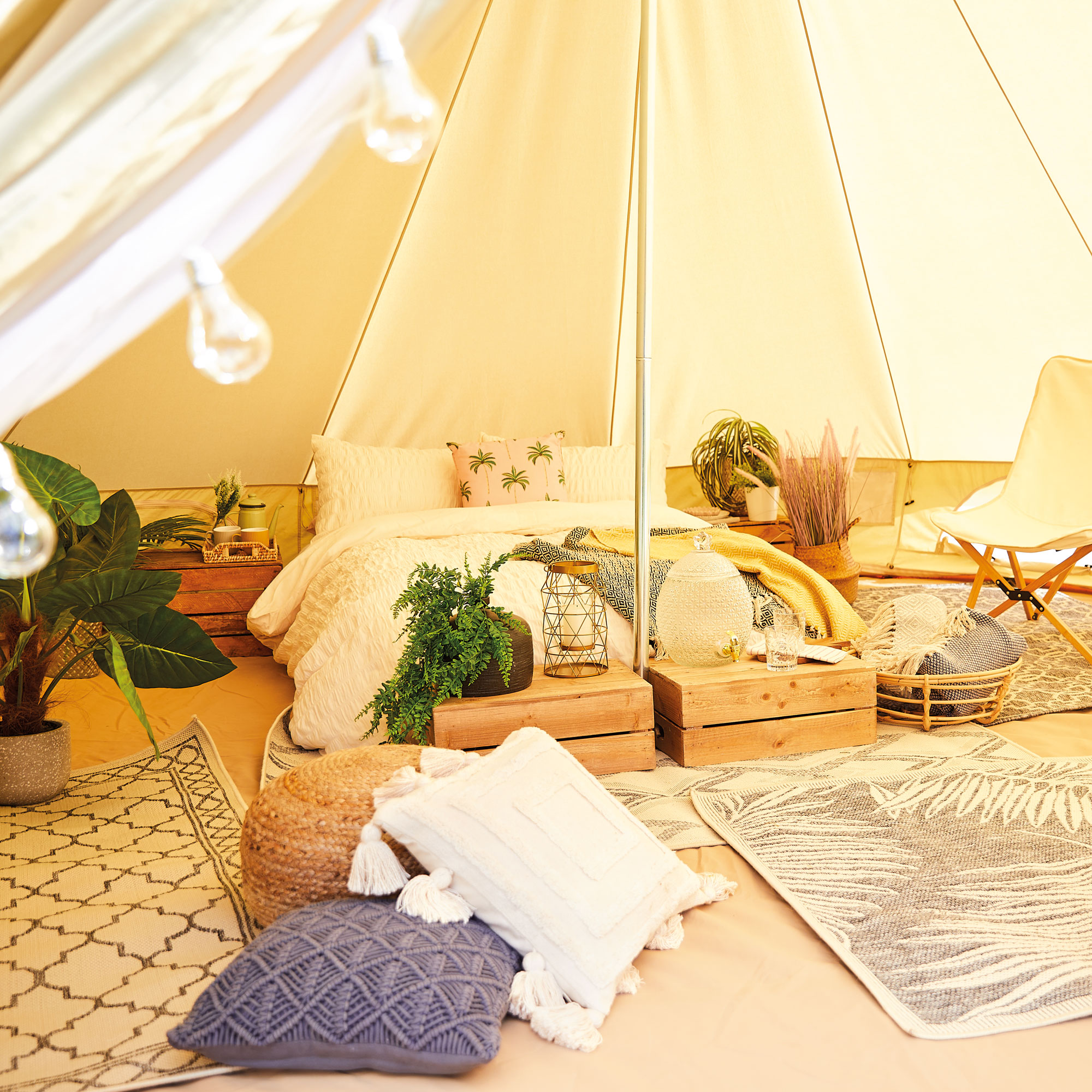The image depicts an inviting interior space inside a tent with a central supporting pole. The white canvas walls slope upwards and are softly illuminated by external light, despite having light bulbs strung along the edges, which remain unlit. The floor is adorned with several monochrome-patterned rugs, primarily in shades of white, grey, and light beige. In the center rests a cozy bed with light beige linens, accented by a yellow blanket and a pillow displaying a green palm leaf print.

In the foreground, various pillows, including a distinctive blue one, are scattered near an oval-shaped dome seat. Two wooden crates serve as makeshift tables in front of the bed, one holding a decorative jar and the other a candle holder. There are also end tables by the bed, each with potted plants adding a touch of greenery to the neutral palette. 

A transparent, lacy curtain drapes from the top of the tent, partially concealing the bed and enhancing the whimsical atmosphere. Contrasting with the predominately white and grey theme, the backdrop features bright orange walls, and the bed itself is positioned on a similarly hued floor. The entire scene evokes a sense of serene comfort, combining natural elements with cozy textiles and thoughtful decorative details.